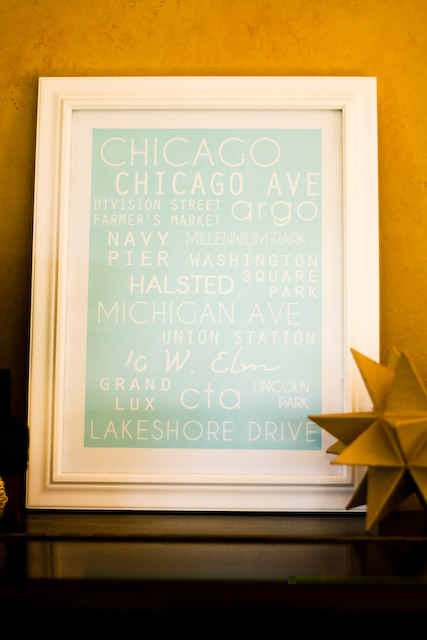The image depicts a framed poster leaning against a yellowish-orange wall. The frame is white with a slight indentation and contains blue or light green background with white text listing various locations: "Chicago, Chicago Avenue, Division Street, Argo, Farmer's Market, Navy Pier, Millennium Park, Washington Square Park, Halsted, Michigan Avenue, Union Station, Grand Lux, CTA, Lincoln Park, Lakeshore Drive, West Elm." To the right of the frame sits a small, dark brown wooden desk adorned with an intricate 3D star-shaped knick-knack with eight triangular sides, adding a decorative element to the scene.